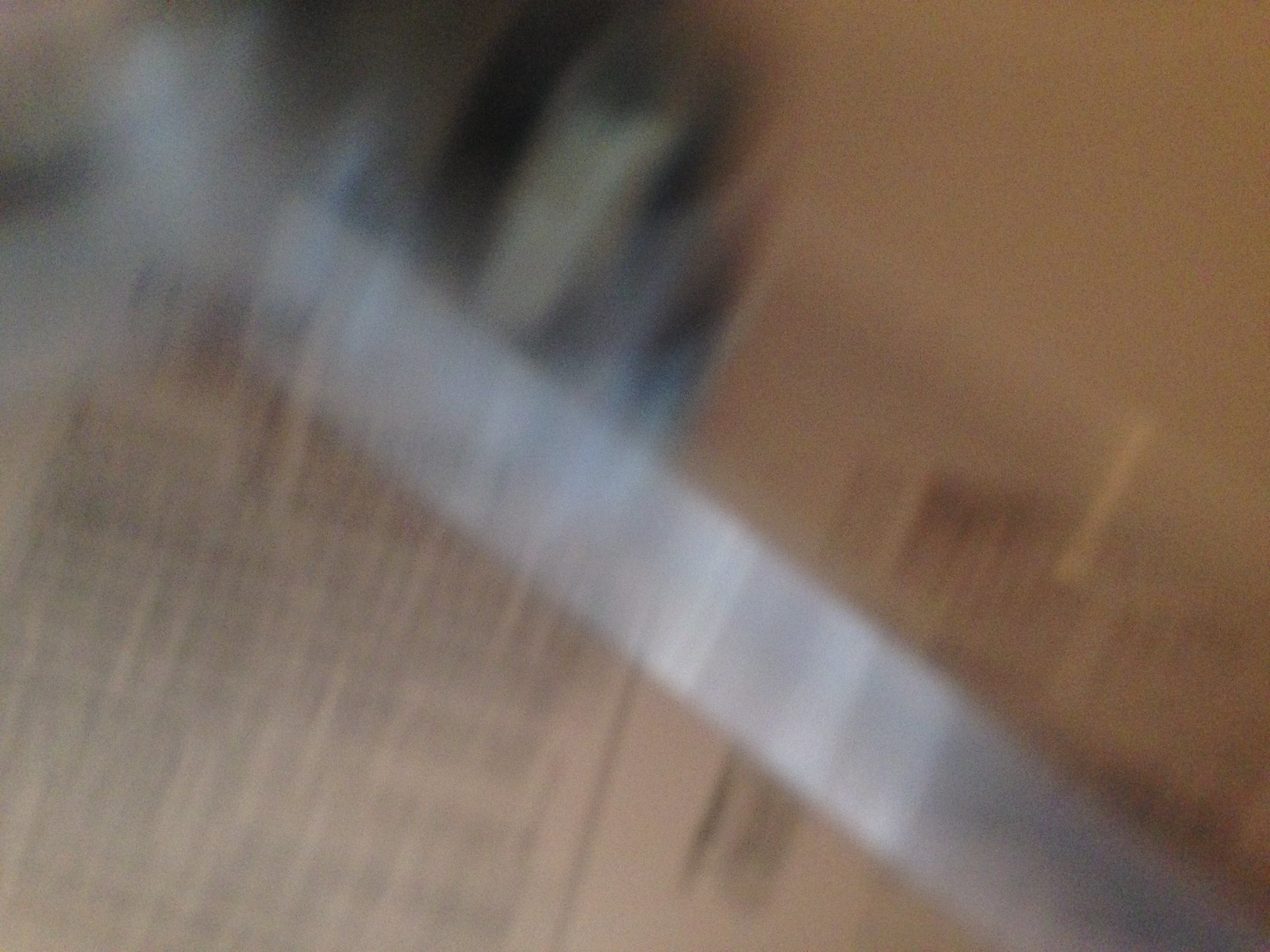The landscape-oriented color photograph is highly blurred, making it difficult to discern specific details. In the top left corner, there's an indistinct series of objects or a multifaceted single object appearing in shades of pale greyish-greeny-blue and darker blue. A white and grayish, pole-like object diagonally traverses the image from top left to bottom right, potentially appearing elongated due to motion blur. Beneath and around these objects, the surface appears to be old newspaper, with slightly yellowed tones and rows of compact, black text in columns, suggesting a faint, closely-cropped section. Hints of bronzy gold can be seen in the top right, with streaks of whitish or silverish-gray possibly being reflections. A faint image in the top center left might resemble a face. Toward the bottom, blurred gray and brown marks provide an unclear background, with hints of brown wood and a less distinct person or face amidst the fuzziness.